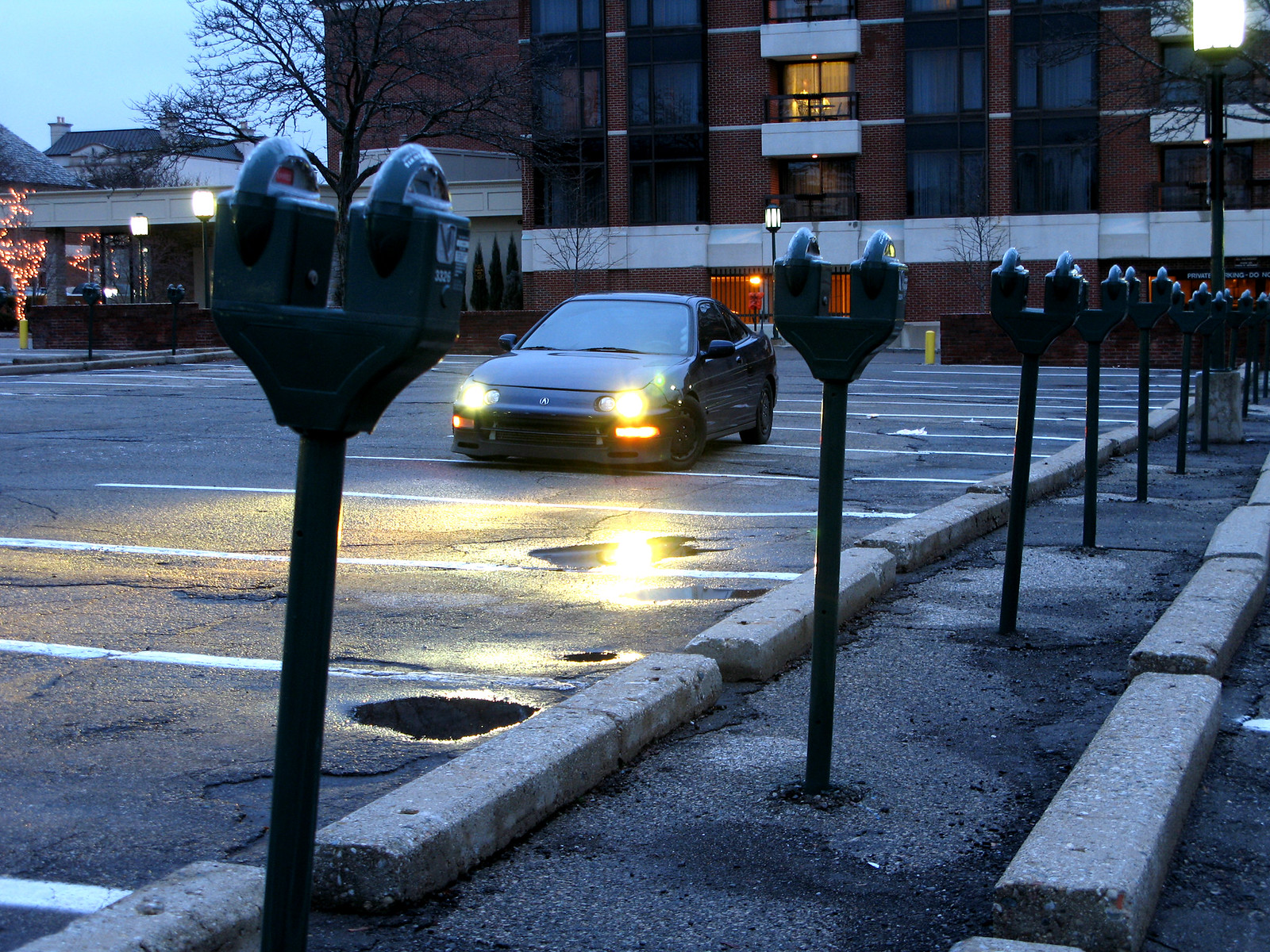This is a color landscape photograph taken at dusk or early evening, capturing a nearly empty urban parking lot. The scene is dominated by a single dark-colored car, possibly from the 1990s or early 2000s, positioned centrally with its yellow headlights on. The car faces the viewer, highlighting the front and side aspects.

The parking lot is defined by white-painted lines marking each parking space, grey cement stops at the end of each space, and a row of parking meters running from the foreground on the left towards the background on the right. The surface is black asphalt. Several street lights and a line of paving stones are visible along the meter row.

In the background stands a red brick building with numerous windows, of which only one is lit up, casting a yellowish glow. There's a white awning along the building's edges and over the windows. Surrounding this building are hints of additional structures, possibly residential condominiums or apartments, with some lit windows and decorative LED lights adorning a leafless tree, adding a wintery ambiance. The sky is a blend of bluish-grey, indicating the transition from day to night. 

The photograph also captures the soft light of the street lamps and showcases silhouettes of trees against the darkening sky, emphasizing the quiet and somewhat solitary feel of the scene.